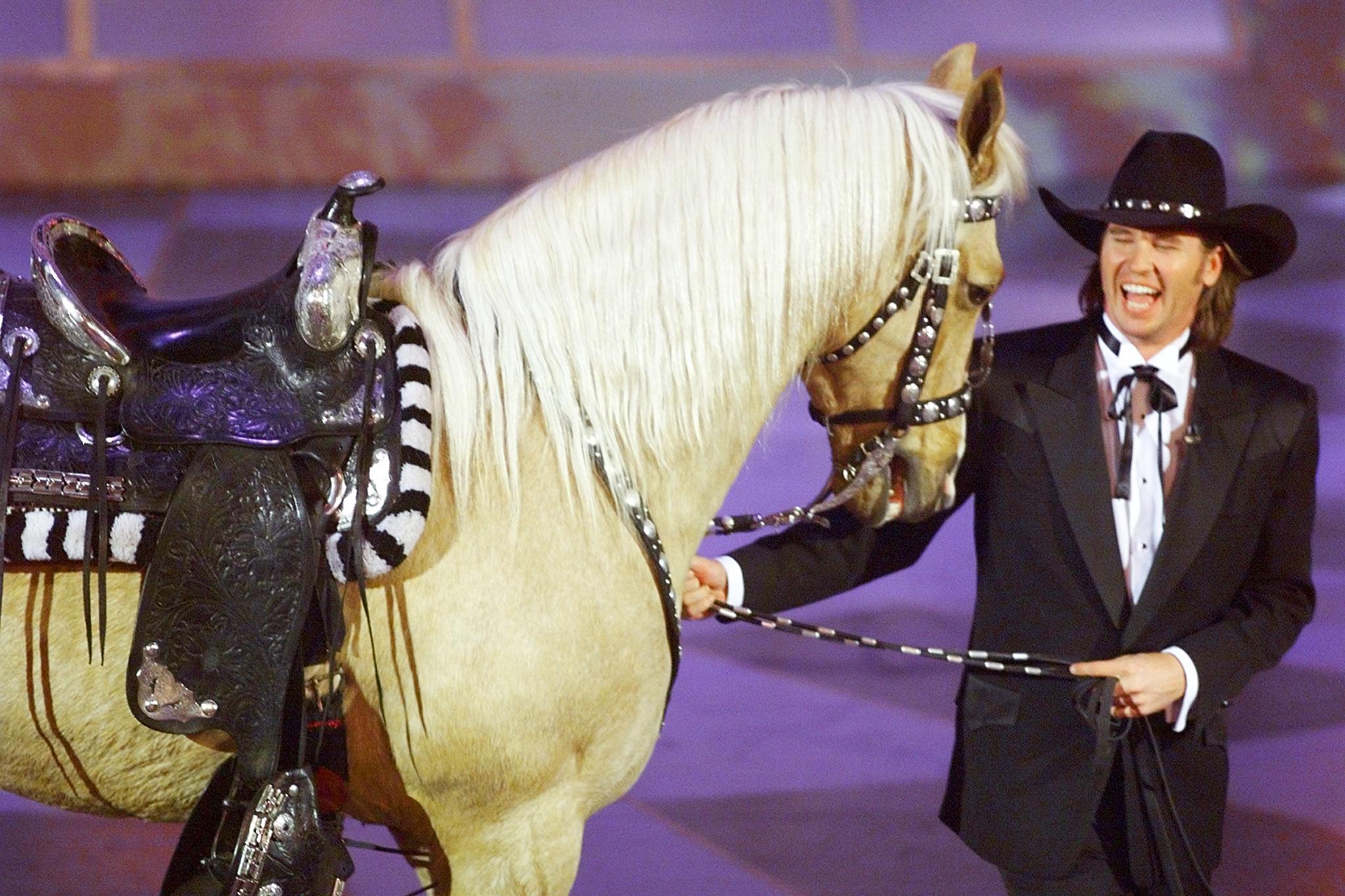In this striking image, Val Kilmer, dressed in an elegant black tuxedo with a white dress shirt featuring dark red accents and a traditional black bowtie, stands confidently on a purple stage. Kilmer’s look is complemented by a black cowboy hat adorned with metallic or jeweled embroidery encircling its base. His long brown hair cascades almost to his shoulders. With his eyes closed and mouth open, he appears to be laughing or perhaps speaking energetically. To his left, he guides a cream-colored horse with a flowing blonde mane and a brown saddle. The reins he holds are a blend of black and white, leading the horse which occupies a significant portion of the image, almost two-thirds. The contrasting colors and elements, from Val Kilmer's Western-inspired attire to the horse’s elegant demeanor, create a compelling and vivid scene.